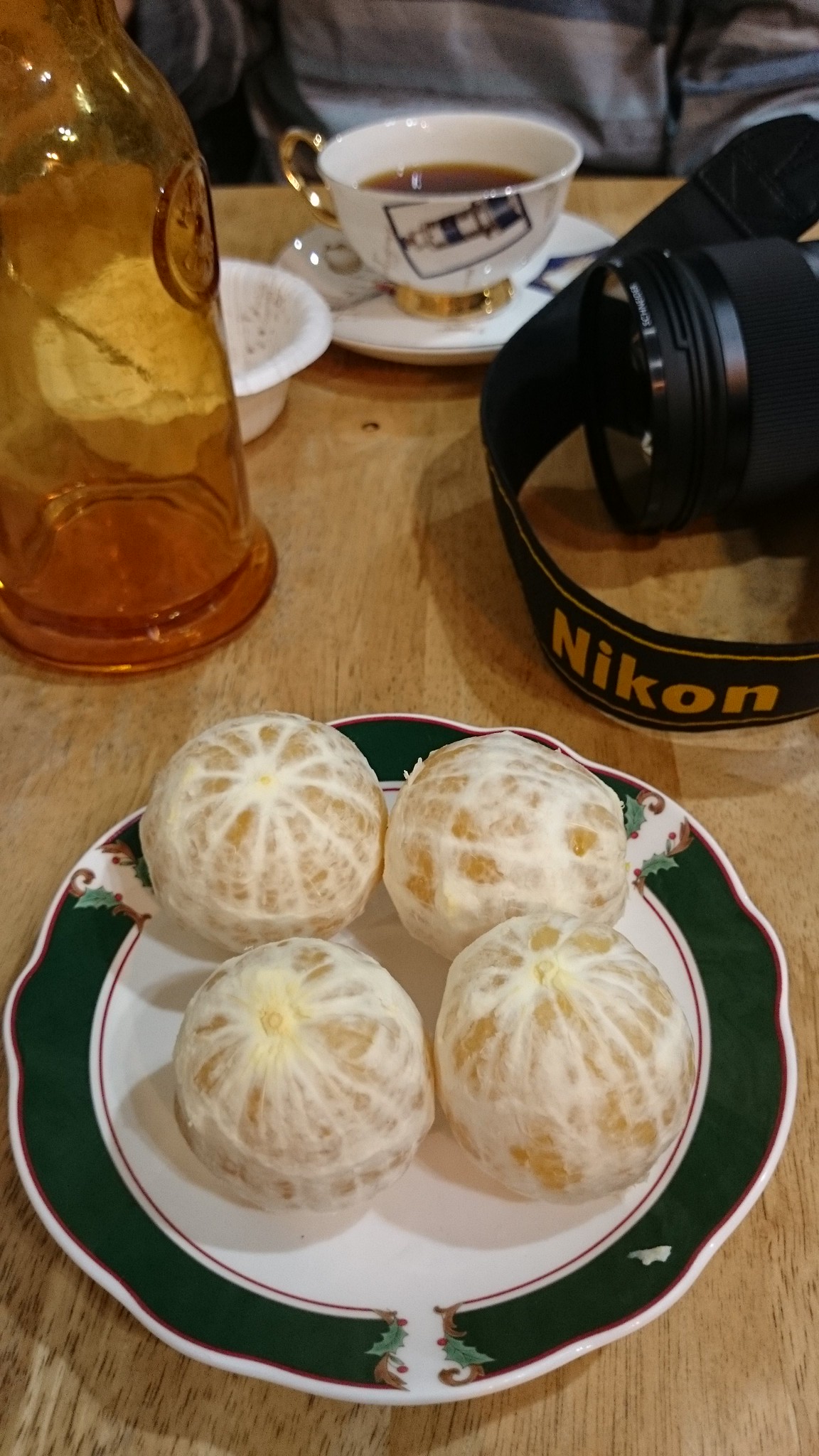This photograph captures a cozy restaurant table setting, taken in portrait orientation with a phone. The most prominent item in the foreground is a black-rimmed plate with a white center, holding four white circular buns with a hint of yellow filling, encased in a delicate spider-like lattice. The plate rests on a weathered light brown table.

On the top right of the image, a Nikon DSLR camera with a distinctive yellow-lettered strap can be seen, pointing towards the viewer. Opposite the camera, on the top left, stands an amber-colored bottle, adding a touch of warmth to the composition.

Across the table, a person clad in a blue-gray sweater is partially visible. In front of them sits a small white cup with a black pattern and gold accents on the handle and foot, likely containing coffee or tea. This cup is placed on a matching saucer. Nearby, there is a white bowl with an indistinct content, accompanied by a utensil, adding to the meal setting. The entire scene exudes a casual, intimate dining atmosphere, rich with details and inviting textures.